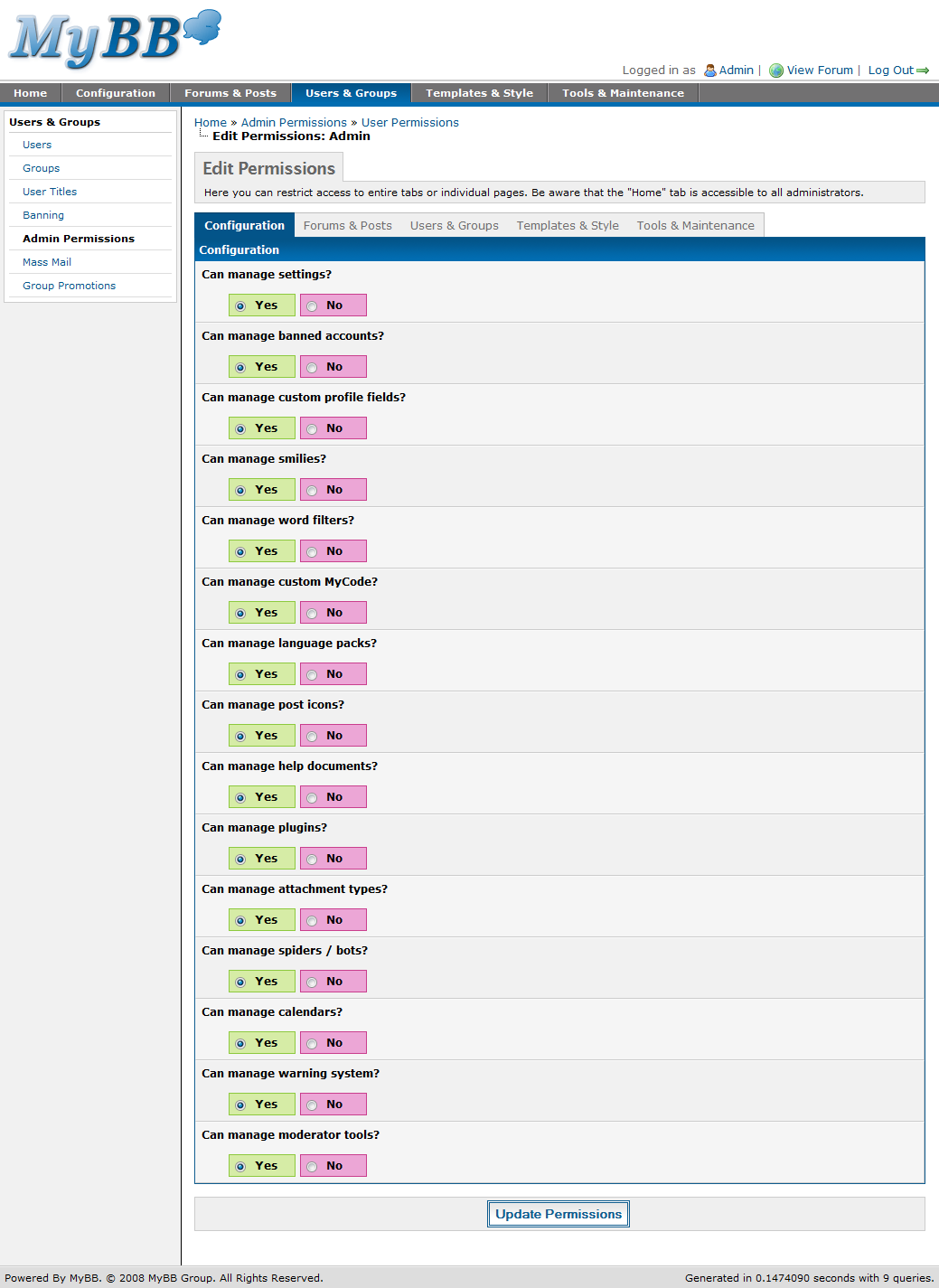This image showcases a screenshot of an online forum administration panel. At the top, the interface displays a white header featuring bold, blue block text in the upper left corner, labeled "my BB," alongside a cloud-like logo to the right. In the upper right corner, the interface indicates that the user is "logged in as admin" with options to "view forum" and "log out."

Below the header is a gray menu banner or line with white text. From left to right, the menu includes options such as "Home," "Configuration," "Forums and Posts," "Users and Groups" (which is highlighted in blue), "Templates and Style," and "Tools and Maintenance."

On the left side of the interface, within a white box, bold black text reads "Users and Groups." Below this, in blue text, are various sub-options: "Users," "Groups," "User Titles," and "Banning." Further down, in black text, it reads "Admin Permissions," followed by additional blue text options labeled "Mass Mail" and "Group Promotions."